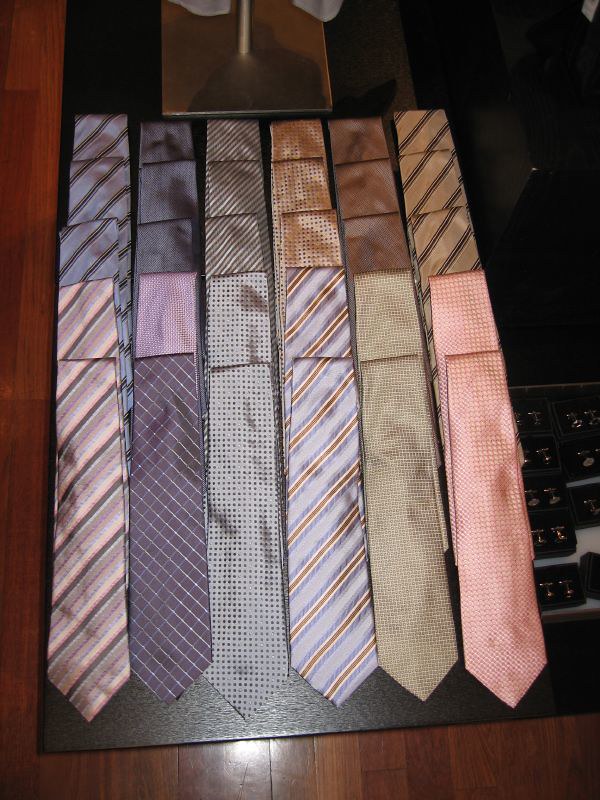This image showcases a neatly organized display of 30 neckties, arranged into six rows with five ties in each row, on a flat surface with a black background. The arrangement appears to be for a shop display rather than a personal collection, as several designs have multiple duplicates.

Starting from the front row, there are three dark blue ties and two tan-colored ties, all featuring stripes. The next row includes three solid black ties, one black tie with a pink pattern, and one black tie with pink stripes. In the third row, three dark green striped ties are followed by two lighter green polka-dot ties. 

The fourth row displays three yellow polka-dot ties alongside two striped ties in light blue and dark yellow. The fifth row has three solid brown ties and two yellow ties with small brown polka dots. Finally, the sixth row contains three dark yellow ties with dark brown stripes and two pink ties adorned with darker pink polka dots.

Adding to the diversity of designs, the collection also includes ties with checkerboard patterns and a variety of color combinations such as black and blue, blue and yellow, silver, and gold with black diagonal stripes. Each tie in this comprehensive array brings a unique style, catering to different pattern and color preferences.